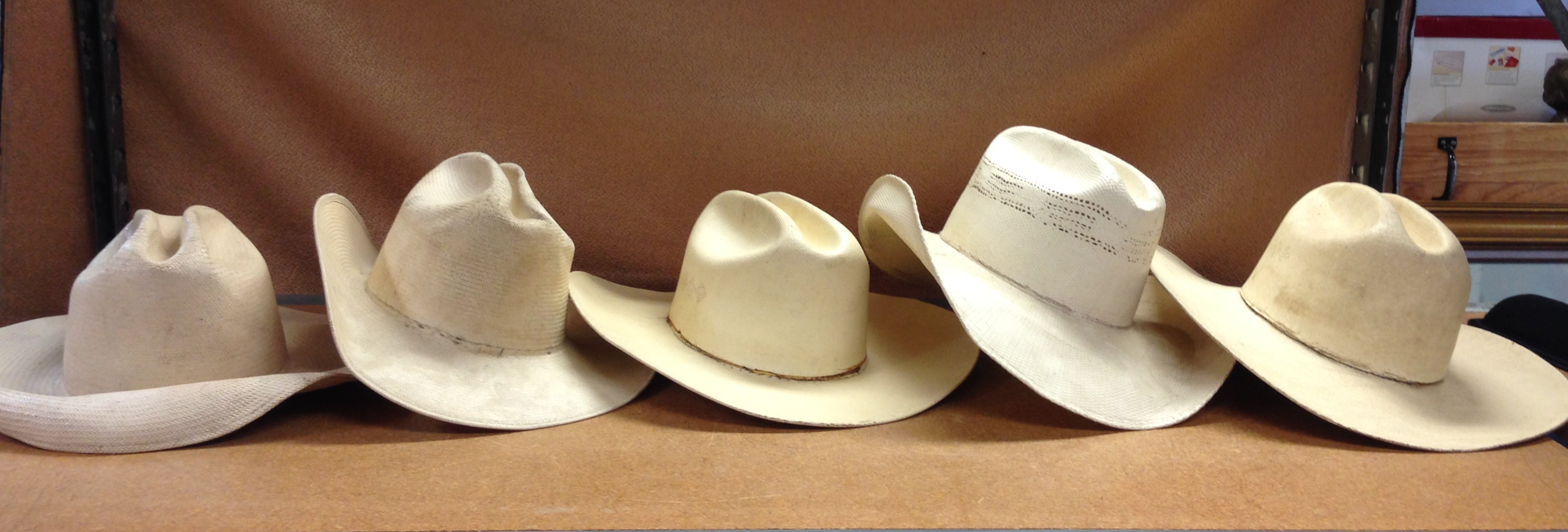The image features five wide-brimmed hats, each varying subtly in shades of light tan and off-white. These hats are arranged in a slightly overlapping line on a wooden table or desk, with a mid-brown curtain serving as the backdrop. The hats are not identical but share small differences in shading, and scuff marks hint at their use. Each hat has a small band near where the brim connects to the head. Notably, the hat in the middle stands out with a slightly different color, and the second hat from the right has some writing or scripture on it. They all have turned-up brims, reminiscent of Stetson or cowboy styles, adding a distinct Western flair to the scene.